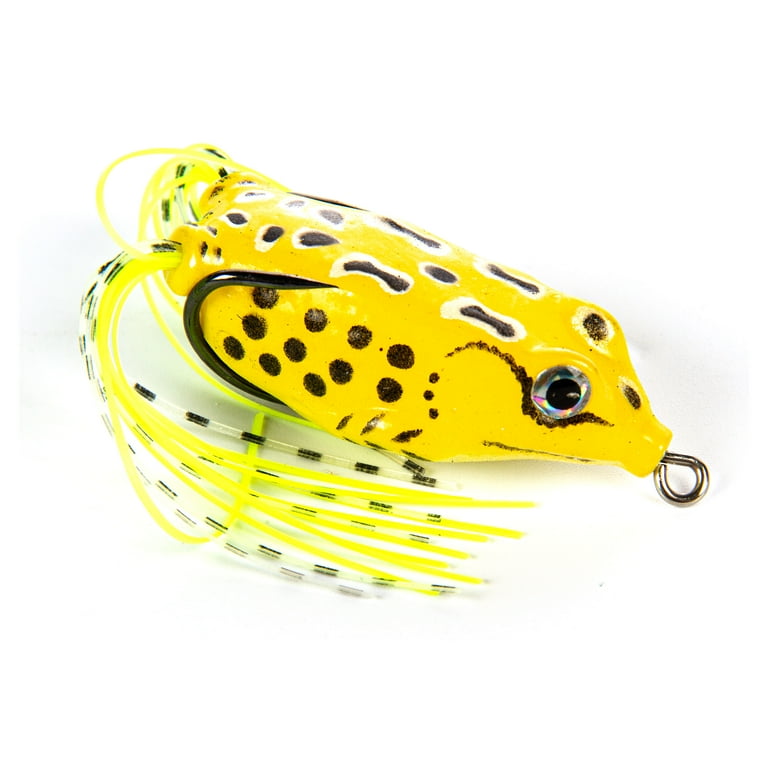This is a close-up picture of a bright yellow fishing lure designed to resemble a small frog. The lure is intricately painted with brown and white dots arranged in frog-like patterns, complete with distinctive googly eyes that enhance its lifelike appearance. Emerging from behind the lure are two sets of yellow streamers interwoven with white and black alternating striped streamers, mimicking the look of frog legs as they move through the water. At the front of the lure is a hook eye for attaching it to a fishing line, while a sharp, steel hook protrudes from the lure's belly, curling up over the back. The background of the image is a plain white, drawing full attention to the detailed craftsmanship and vivid colors of the lure.